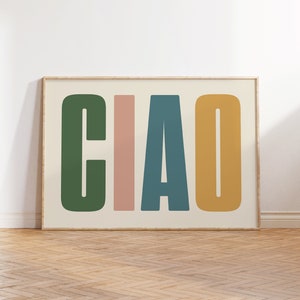The image depicts a framed poster featuring the word "Ciao," framed by a thin, tan wood frame. It is leaning against a white wall and sits on a tiled floor with a light to medium brown, zigzag wood pattern. The floor tiles appear somewhat unclean. The frame is rectangular and houses a white background with four large, colorful block letters: C in dark green, I in dark pink, A in dark blue, and O in a light brown or tan color. The scene is well-lit, possibly from sunlight coming in from the right side, casting shadows on the left. There are no other objects, people, or text in the photo, and a white baseboard is visible at the bottom of the wall.